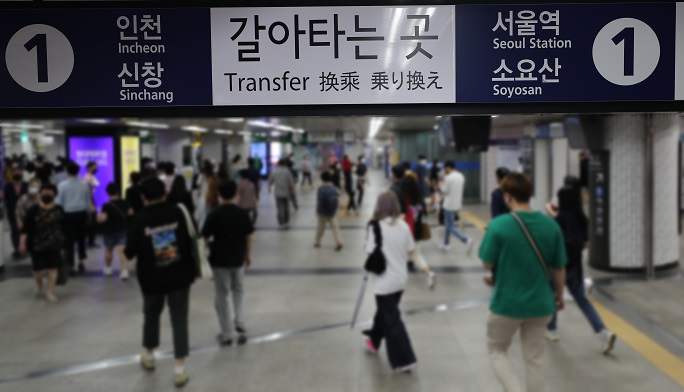The image depicts a bustling scene at Seoul Station's underground subway platform, presumably in South Korea, where numerous people, including men, women, and children, are traversing through the area. Prominent above the crowd is a large sign displaying the number "1" alongside station names in both Korean and English: "Incheon" and "Sinchang" to the left, "Seoul Station" and "Soyo Sanso" to the right. The sign also features the word "Transfer" and includes additional Chinese characters. Multiple individuals, some donning masks, navigate the subway environment marked by a yellow safety line, various pillars, and visible LED signs. The attire of the subway-goers ranges from green shirts and khaki pants to white shirts with black pants, as well as black and gray clothing combinations. The scene is a vivid snapshot of the diverse public making their way through the extensive and busy subway system.